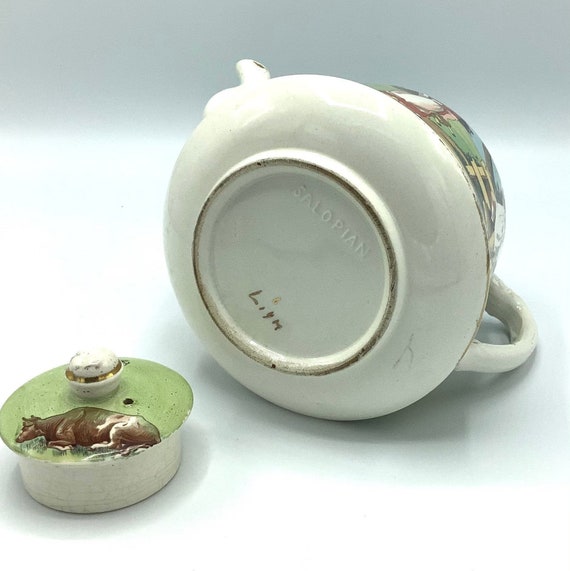This photograph captures a detailed close-up of an antique Limoges teapot, positioned on its side to prominently showcase the branding and signature on the underside. The teapot, likely a sale item, rests on what appears to be a white surface against a light gray background, giving it a clean and professional presentation. The teapot's bottom displays the inscription "Limoges" and what seems to be the painter’s signature "L-I-G-M," along with the brand name "Salopayan." 

Adjacent to the teapot lies its matching green lid, which is topped with a raised, intricately painted brown cow lying down, evoking a pastoral scene. The lid also features a distinctive gold ring on the knob, complementing its light green hue. Additional details, like the silver-rimmed top of the teapot and its handle, underscore the craftsmanship of this ceramic piece, hinting at its potential historical and monetary value. The meticulous arrangement and clarity of the image suggest it is intended for showcasing the teapot's features, possibly for sale.